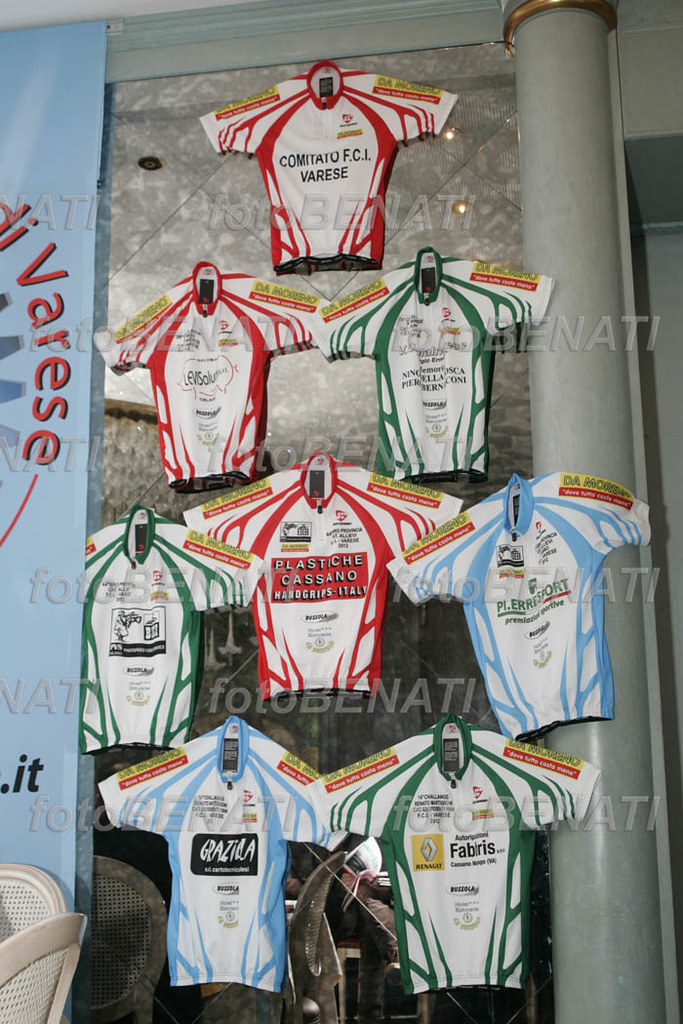This image captures a store window display featuring various jerseys, potentially for a biking or racing team. The photograph is overlaid with a tiled watermark that says "FOTOBENATI," spelled F-O-T-O in lowercase and B-E-N-A-T-I in uppercase, in a faint gray color. In total, there are eight jerseys arranged on a wall in rows: one at the top, two in the second row, three in the third row, and two in the bottom row. These predominantly white jerseys have different highlighted colors: the top one is red, the next row includes one red and one green, the third row features green, red, and blue, and the bottom row has blue and green. 

Various writings and logos are visible on the jerseys, suggesting sponsorships or affiliations. The top red and white jersey bears the name "Camito F.C.I Varese," another mentions "Lewis Solutions," and another reads "Plastiche Cassano Hand Grips Italy." A light blue banner with red text spelling out "VARESE" hangs on the left-hand side of the display. Additional elements in the image include the corner of a white chair in the bottom left and a pole coming down the right side of the display. The background features a glass pane with a marble-like appearance.